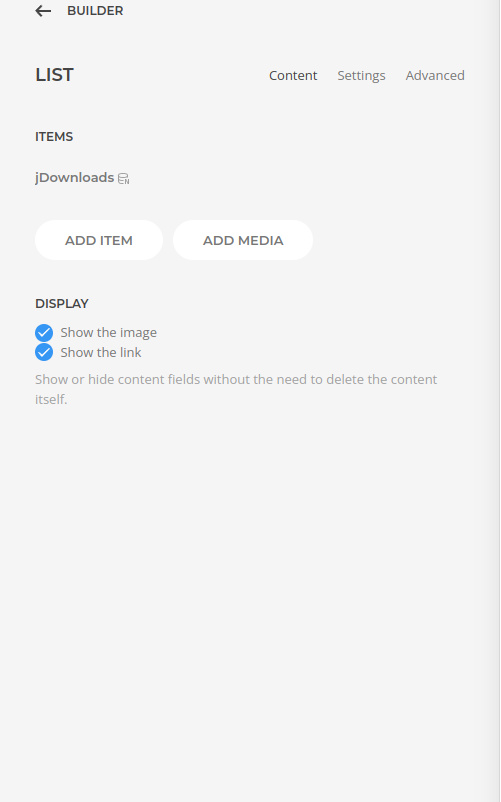This is a detailed screen capture of a settings section, likely from an application or website, with a light gray background. The right-hand side features a subtly rounded, darker edge that transitions into the lighter gray. At the top left, there is an arrow pointing left next to the word "Builder." All text is in a dark gray shade, not quite black.

Adjacent to the word "Builder," there are three links: "Content," "Settings," and "Advanced," with "Content" being the currently selected option, highlighted in a darker shade than the others. Below these links, in bold text, the word "Items" is displayed, followed by "J Downloads" and a small symbol that appears to feature the letter "N," possibly a logo or an icon.

Further down are two rounded white buttons with gray text labeled "Add Item" and "Add Media." Below these buttons, another bold heading reads "Display." Here, two round circles with white check marks are visible, labeled "Show Link" and "Show the Image." Directly underneath, a description reads: "Show or hide content fields without the need to delete the content itself."